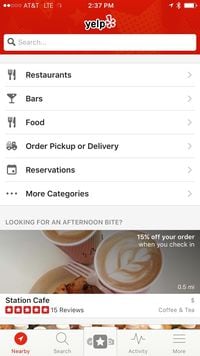The image appears to be a screenshot from a smartphone, displaying the user interface of the Yelp app. At the very top of the screen, there is a status bar featuring a red background. In the upper left corner, five circles are shown, with the first two filled white. To the right of these circles, the carrier information "AT&T" and the connectivity status "LTE" are visible. Centered in the status bar, the time is displayed as "2:37 p.m." On the far right, a mostly filled battery icon indicates ample remaining battery life.

Beneath the status bar, the word "Yelp" is prominently displayed in black text in the middle of the screen, accompanied by a large white search bar directly below it. Following this section, six navigational options are presented. The first option reads "Restaurants," paired with a fork and knife icon. The second option, labeled "Bars," is represented by a martini glass icon. The third option, "Food," also features a fork and knife icon. Next is "Order Pickup or Delivery," indicated by a car icon, followed by "Reservations," denoted by a bag icon. The final option includes three dots and the text "More Categories."

Further down the screen is a rectangular section containing an image. This image shows a cup of coffee decorated with a series of hearts, accompanied by a plate of food with a white plastic fork. In the upper right corner of this image, text announces "15% off your order when you check in." Below the image, the text "Station Cafe" is displayed, followed by a five-star rating and the note "15 reviews."